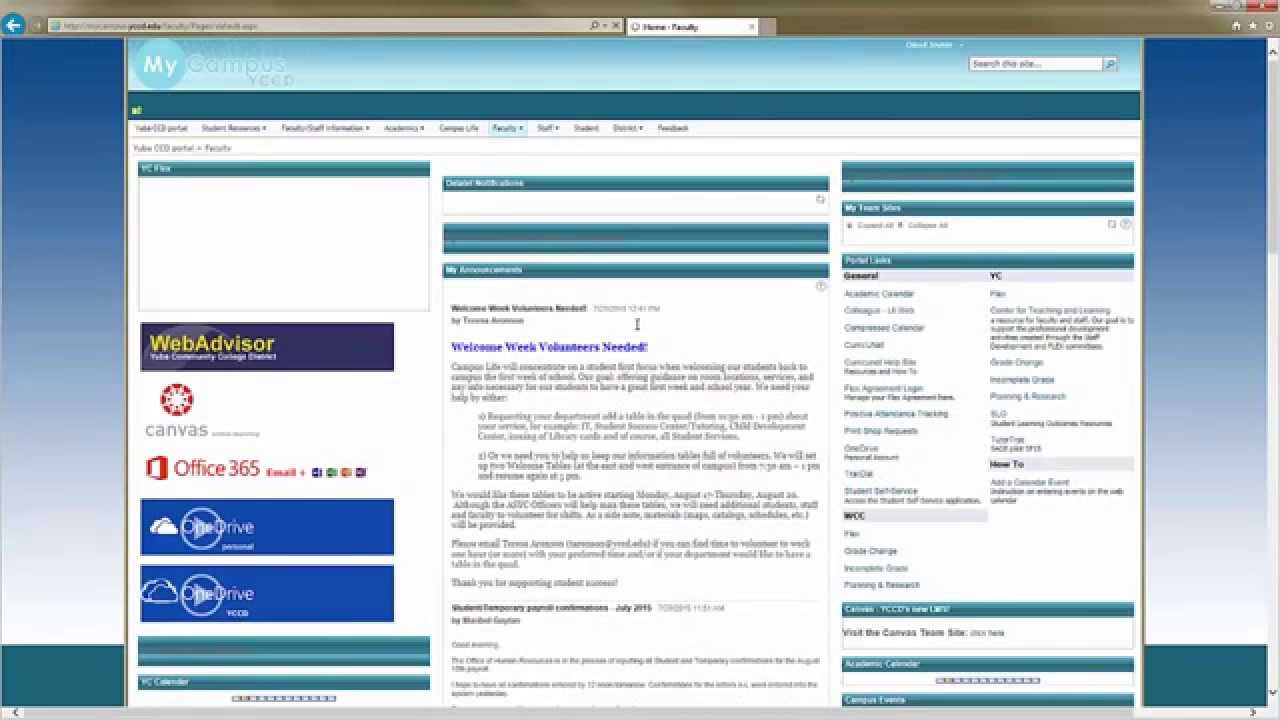This image is a computer screenshot displaying a complex interface adorned with various graphical elements and text. At the top of the image, there is a gray bar featuring a search item, which is followed by a predominantly white screen bordered by shades of blue on each side. The blue color gradient transitions from darker blue to gray, eventually fading into a lighter gray. Towards the bottom of the image, on either side of the main portion of the screen, there is a teal-colored bar, framing the central content which is enclosed within a white screen outlined in black.

At the top of this central white screen, there is a light blue bar. On the left-hand side of this bar, there is a circular icon containing the letters "MI" and accompanied by the word "campus". On the right-hand side of the top bar, a search bar is situated. Below this, there is a dark green bar with categorized headings listed beneath it.

Further down, the central area of the layout includes a white box on the right-hand side, topped by a green bar. Within this white box, the words "WebAdvisor" are displayed in yellow font against a black background, followed by "Canvas Office 365". Below these items, several blue bars are labeled "OneDrive". Two green lines are positioned under these elements.

In the core section, three green bars are present with the text "Welcome, week volunteers needed" prominently displayed. Shifting attention to the right-hand side of the image, two green bars are seen, followed by a search bar and another green bar. Additional information is included under a section titled "General Information," listing various items. Towards the bottom, another green bar appears, succeeded by additional text, another green bar, a white space, and yet another green bar situated at the very lowest part of the image.